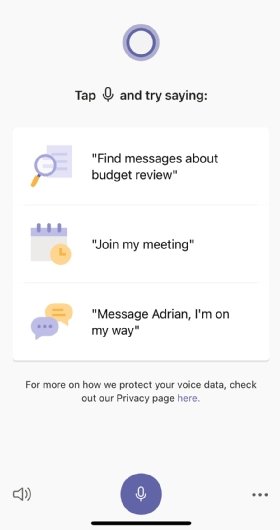At the top of the image is a blue circle with a clear interior, approximately two inches in height. Below this circle, black text reads "tap," accompanied by an icon of a speaker symbolizing a microphone. Following this, the text "try saying:" is presented, leading to an icon of a magnifying glass in front of a piece of paper. Next to this icon, the text reads "find messages about budget review," all enclosed in quotations.

About two inches further down, there is an icon of a calendar with a clock positioned in front of it. Beneath this visual, the printed instruction or quoted text reads "join my meeting." Adjacent to this are two speech bubble icons—one purple and the other yellow—enclosed within quotation marks with the example text: "message Adrian I'm on my way."

Continuing downward, black text states: "For more on how we protect your voice data, check out our privacy page here." The word "here" is rendered in light gray, indicating it is a clickable link.

At the very bottom left of the image, there is an icon of a speaker emitting circular lines, and next to it, an icon of a microphone housed within a purple circle, roughly two inches in diameter.